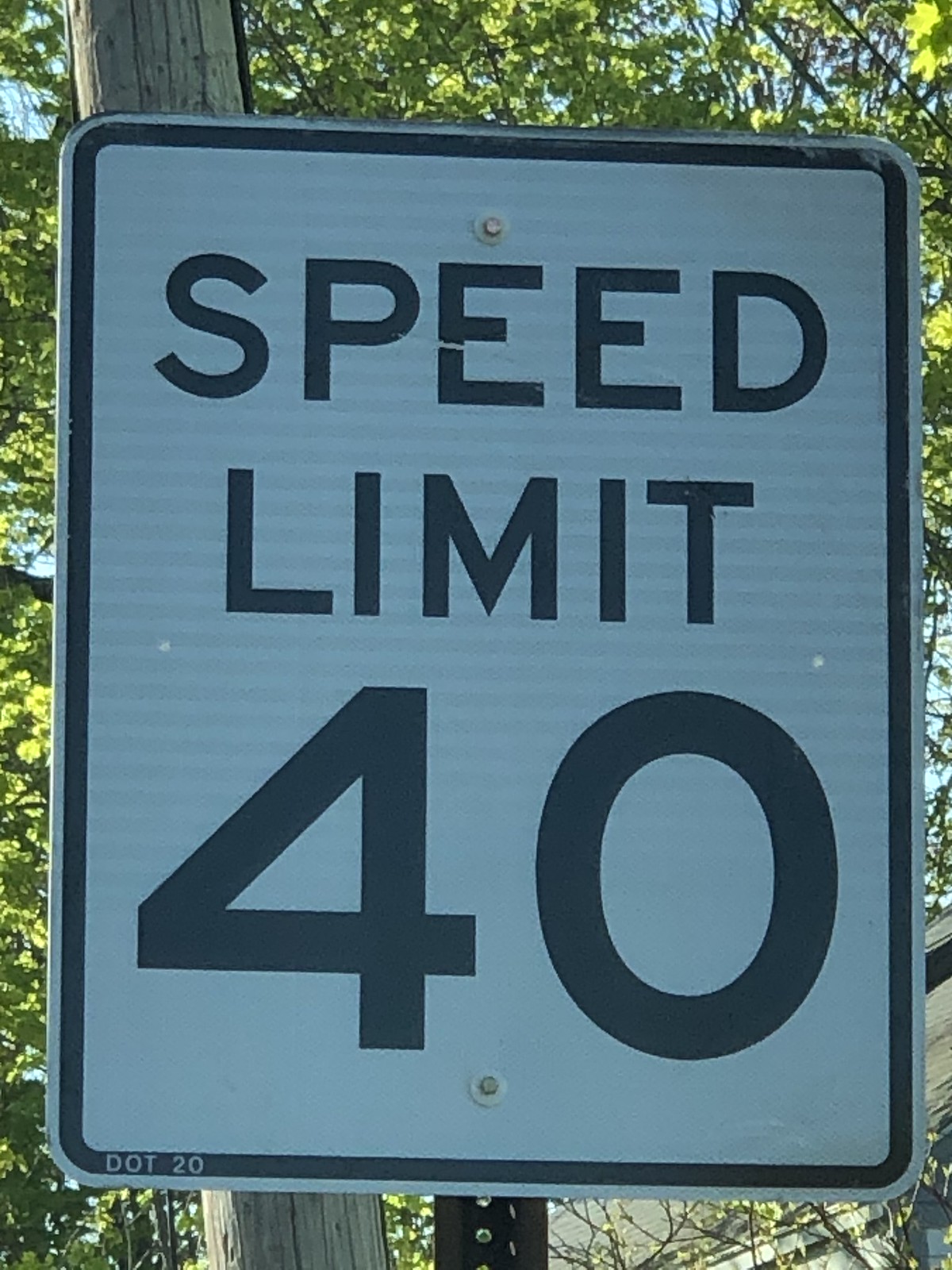In the photograph, we see a close-up image of a speed limit sign set against an outdoor backdrop. The white (appearing somewhat gray due to shadow) aluminum sign prominently displays in bold black text "SPEED LIMIT 40" with a black border. The lower left corner also bears the marking "DOT 20." The sign is affixed to a perforated metal post, partially visible at the bottom of the image along with the mounting bolts. In the background, there’s a faint view of what seems to be a gray telephone or power line pole, complemented by green tree leaves. Patches of blue sky peek through the foliage, adding depth and color contrast to the scene.